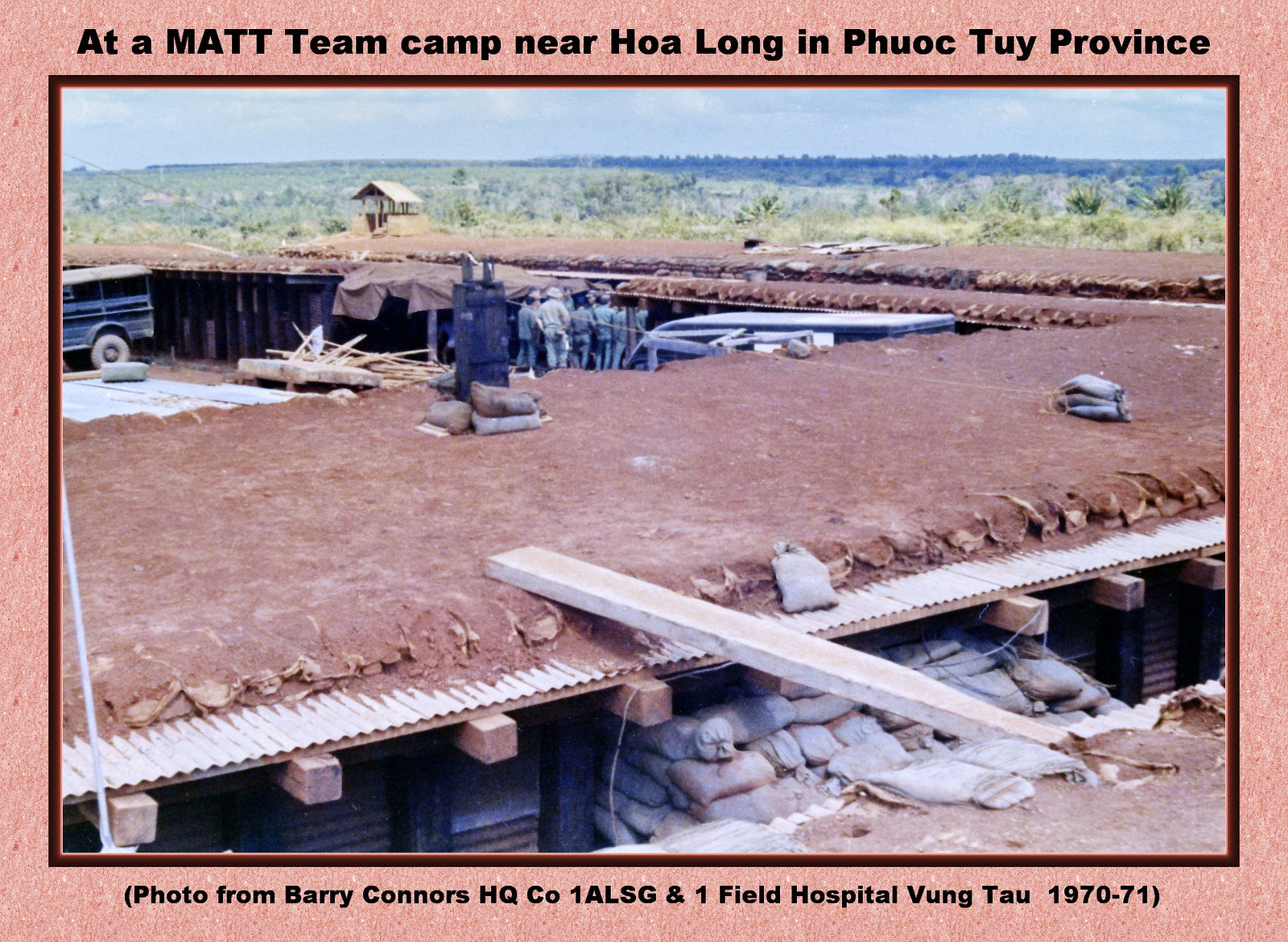This outdoor color photo depicts a construction site at a MAT team camp near Hoa Long in Phuoc Thoi province, as per the caption, with the photo credited to Barry Connors from the HQ Co-1 LSG and one Field Hospital in Vung Tau, dated 1970-71. Central to the image is a building excavated into the ground with a dirt rooftop. A wooden plank bridges this rooftop to another similar structure, with sandbags placed strategically between them, likely for stability. In the background, more of these underground structures are visible along with a grassy area featuring a house and a blue vehicle. Approximately twelve men stand in front of one of these structures, appearing to gather and prepare for their work.